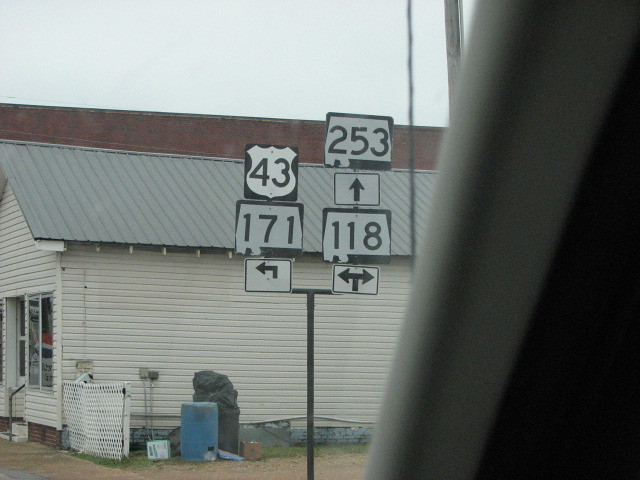This photograph captures a unique street sign arrangement viewed through a windshield. Centered in the image, a black metal pole splits into two horizontal arms. On the left arm, three distinct signs are displayed: a small white rectangle with a leftward arrow, a black square partially bordered in black indicating "171," and above them, a black sign featuring a white shield with the number "43." To the right arm, the signs include a white background with a black double arrow pointing left and right, a square sign edged in black reading "118," and above that, a square white sign with an upward arrow displaying "253." The backdrop features a white one-story building with a dark gray roof, visible meters, a portion of a white fence, and a blue, slightly worn trash can on the side.